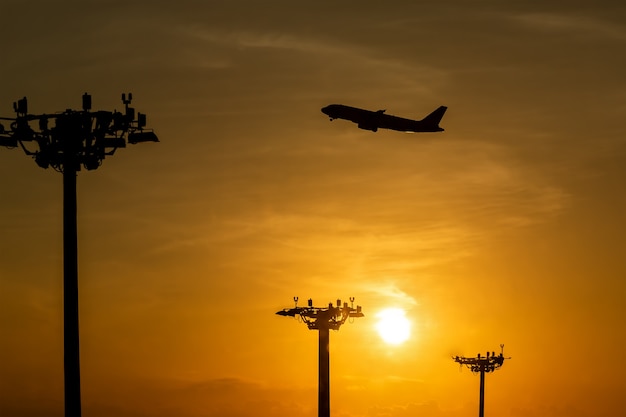In this captivating photograph, we see the striking silhouette of a large passenger jet taking off from an airport, captured against an amber sky where a white sun is either setting or rising. The airplane is almost entirely black, with its front wheel partially enclosed as the landing gear is lifted. Positioned centrally towards the upper portion of the image, the jet ascends from right to left. Below and starting from the center left, extending diagonally to the bottom right, are a series of runway lighting towers. These towers, equipped with transmitters and directory assistance, stand tall and progressively diminish in size as they move into the distance, marking the landing pattern. The sky is a blend of light and dark oranges, creating an enchanting forest perspective ambiance. The scene combines the stillness of the twilight sky with the dynamic energy of the aircraft in motion, silhouetted against the radiant backdrop.